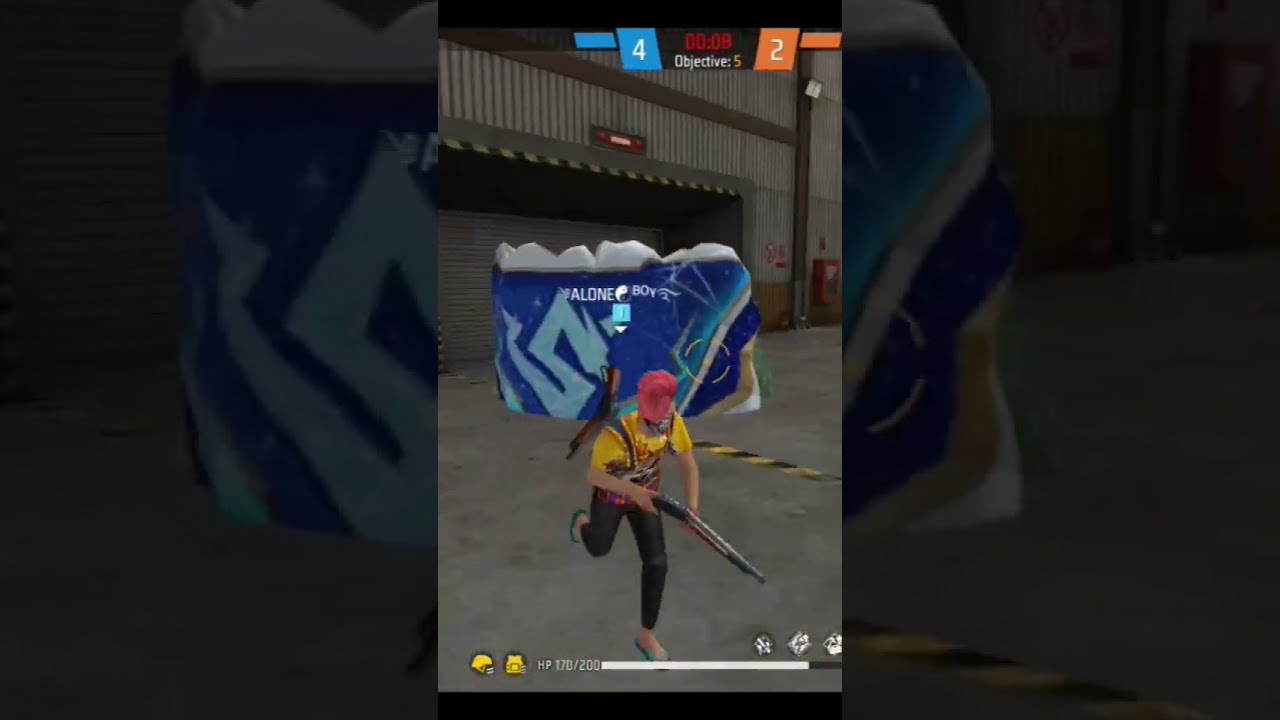In this detailed screenshot from a video game, we see the main character prominently featured in the center of the image, which appears to be presented in a vertical, portrait-like format. The character is dressed in a yellow shirt, black pants with black suspenders, and green sandals. He is also wearing a red cap and a red mask that obscures his face. He's armed with a shotgun in his hands and has another sawed-off shotgun strapped to his shoulder. The character is running downwards and to the left, seemingly towards the viewer.

The backdrop displays what looks like a street or a room, dimly lit, with a dark gray building or structure behind him. There is a damaged advertising sign or a piece of a large blue tarp behind the character, featuring a light blue "S" and various shades of blue, with signs of wear and graffiti. This object appears to have fallen or been damaged, possibly relating to a warehouse or closed shopping center setting. 

On the ground, there's a black and white striped road marking. The overall scene suggests an urban environment, possibly post-apocalyptic or in the midst of some chaotic event, hinting at a zombie or survival scenario.

In terms of game interface, at the top of the image, a match score is displayed with an objective status showing "Objective: 5." There are two colored boxes - a blue one with a score of 4 and an orange one with a score of 2, both labeled with white numbers. Additionally, a countdown clock indicates there are 8 seconds left in the current objective. At the bottom of the screen, a hit points bar provides vital information for in-game status and player health.